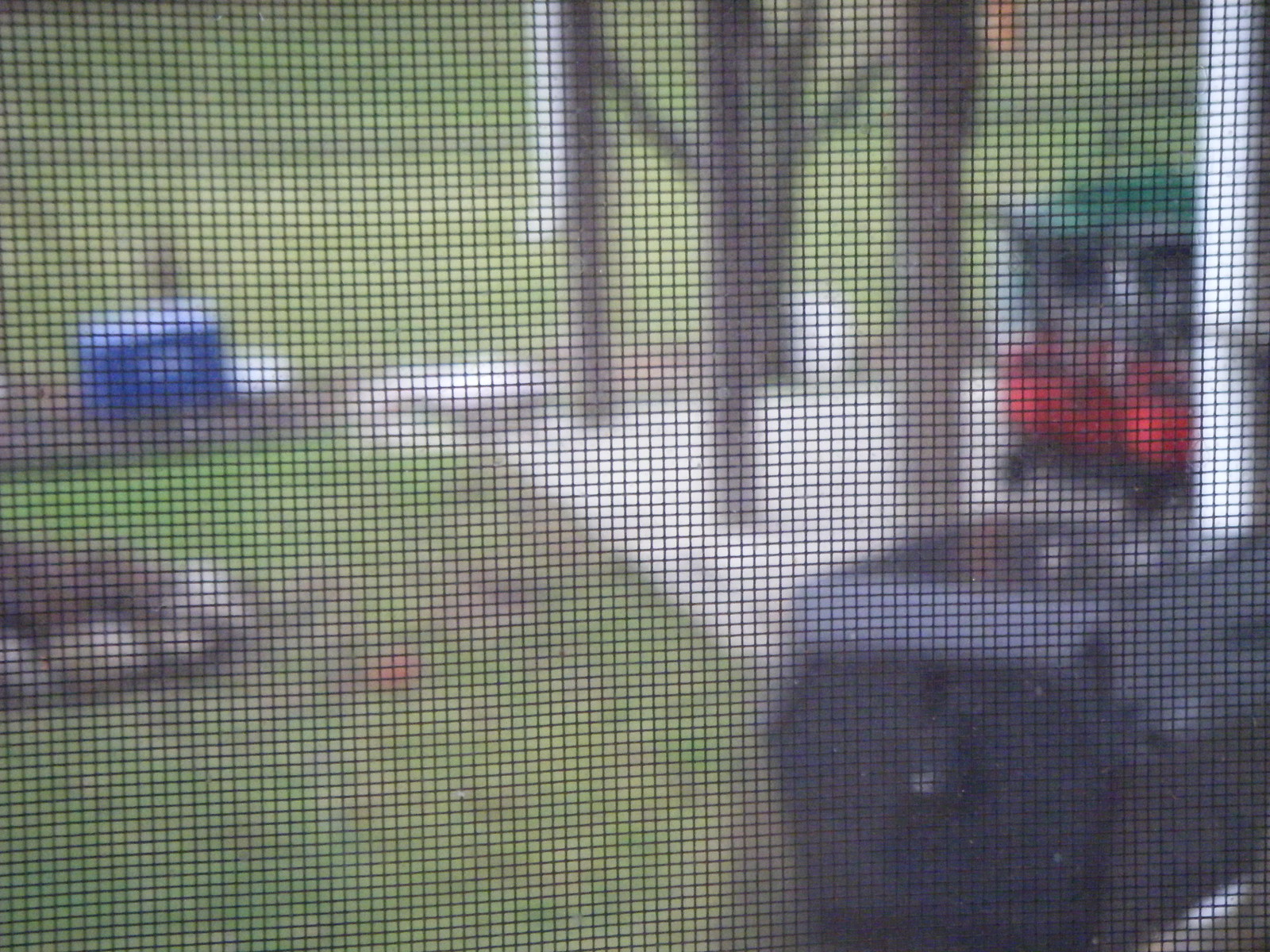This is a blurry photograph taken from behind a mesh screen, capturing an outdoor area possibly viewed from a home patio. The mesh grid partially obscures the view, but several elements are distinguishable. At the forefront, there is a barbecue grill situated in front of the mesh. To the left side of the yard, a rock enclosure, potentially a fire pit, can be seen with some stones arranged in a circle. Nearby, there's a tall wooden frame structure that resembles an upper deck, supported by three substantial beams emerging from a grey concrete base. Further into the yard, a blue and white cooler sits on a brown surface, possibly dirt. Additionally, there's a green and red children's toy car with wheels visible. The yard appears well-maintained with a healthy spread of green grass, bathed in daylight, likely in the early afternoon between 1 and 4 p.m.